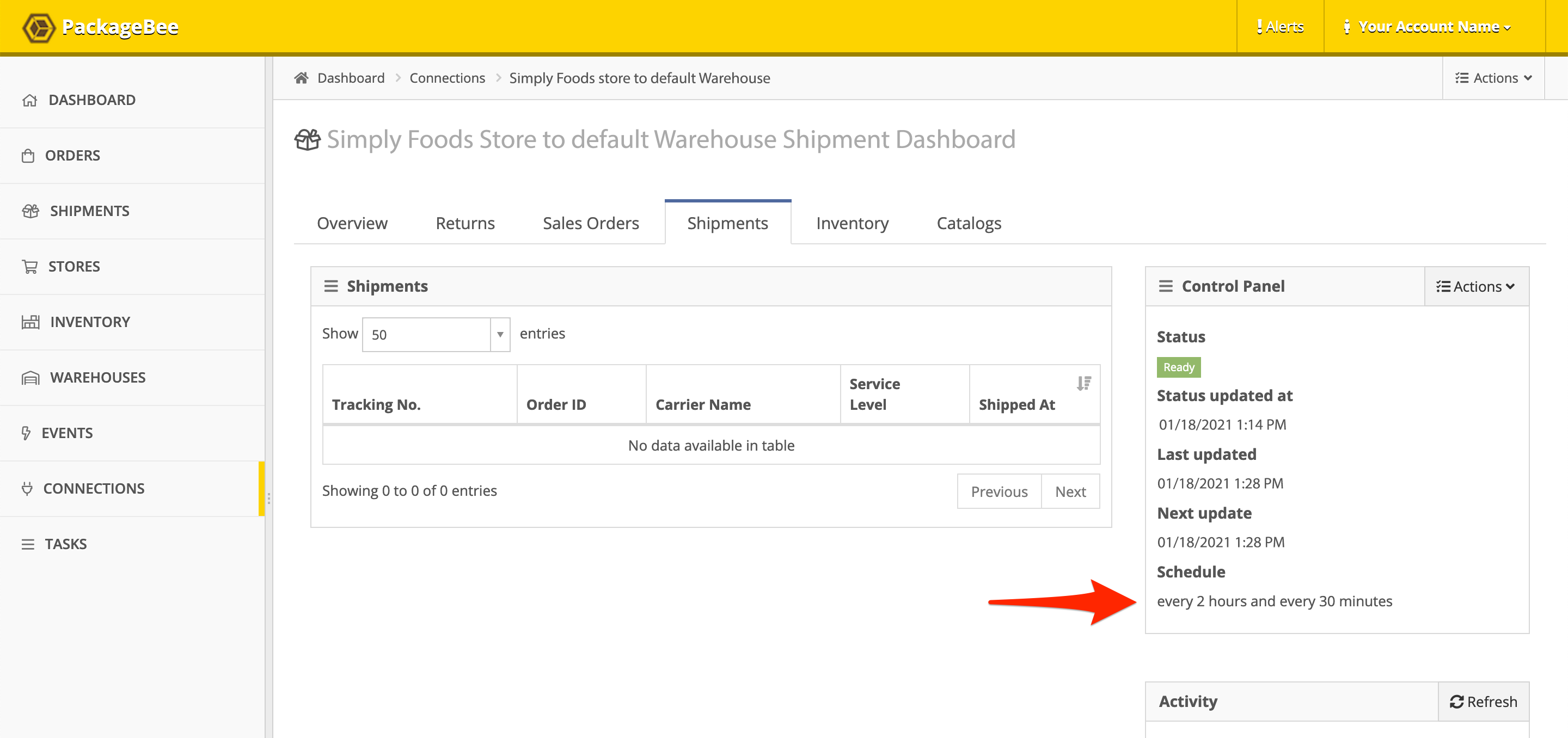The image depicts a logistics management interface from a platform referred to as "Package B." The screen is divided into two main sections: a navigation pane on the left, and a larger main section on the right. In the left pane, a list of options is visible, including Dashboard, Orders, Shipments, Stores, Inventory, Warehouses, Events, Connections, and Tasks. The user has selected "Connections" from this list.

The main section displays details regarding the "Simply Foods" store and its connection to the default warehouse shipping dashboard. This interface appears to focus on various aspects of logistics management. Several tabs are visible near the top of the main section, labeled Overview, Return Shipments, Sales Orders, Inventory, and Catalogs. The "Shipments" tab is currently active, which reveals that there are no shipments listed at this time.

To the right of these tabs, a control panel labeled "Status: Ready" is shown. The status was last updated on June 18th, 2021. The image includes a red arrow pointing to a specific area within this control panel, highlighting settings that specify a scheduled update every two hours and every 30 minutes.